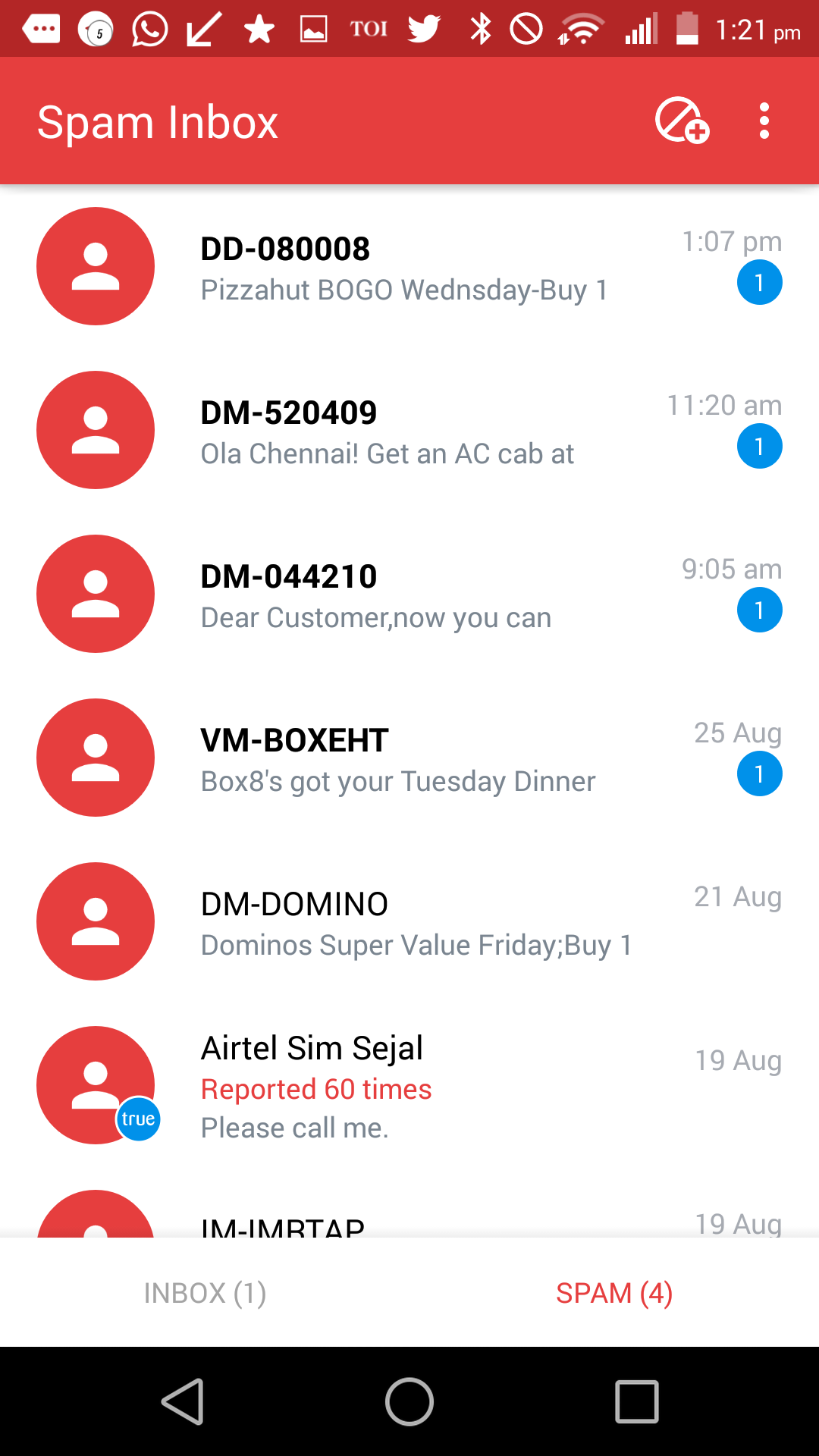The image is a screenshot of a mobile device's screen captured at 1:21 PM, as indicated by the time displayed in the top right corner. The status bar at the top showcases a series of icons, including WhatsApp, Gallery, Twitter, the Bluetooth icon, the Do Not Disturb icon, and the Wi-Fi signal strength showing 3 out of 4 bars. Additionally, the network signal strength is strong with 4-5 bars, and the battery level indicator is also present. 

Significant notifications include messages in the spam inbox from "dd-080008," "dm5-520409," "hola chanel," and a note about getting an AC cab out. Specific contacts listed are Etel Singh and Sergio, who has been reported 60 times, along with a message requesting a call back.

The main portion of the screen features an inbox with 1 message and a spam folder containing 4 messages. At the bottom, the legacy Android navigation keys are visible, which include the back button, the menu button, the home button, and the recent apps key. Dominant colors in the image are red, white, and blue. There is also a promotional message from "dm-domino" advertising Domino's Super Value Friday deal, offering to buy one item.